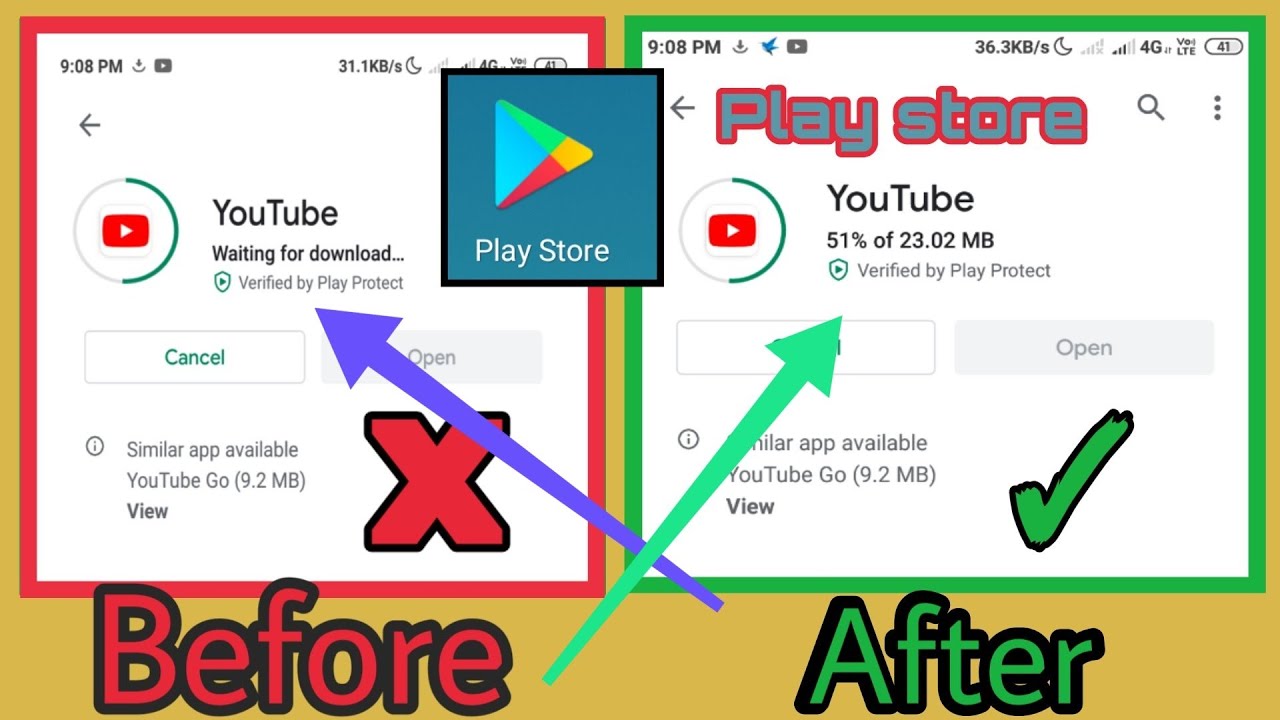This image is a step-by-step tutorial demonstrating the process of downloading the YouTube app from the Google Play Store. The entire composition is set against a mustard yellow background.

**Left Screenshot (Before):**
- The left side features a screenshot outlined in a thick red line, displaying the initial stage of the download process.
- At the top of the screen, the time reads 9:08 PM, along with download, signal strength, and battery status icons.
- The main content shows the YouTube logo within a circle, followed by the text "YouTube" and "Waiting for download." 
- A purple arrow points from the bottom right corner to the text "Verified by Play Protect," emphasizing this status.
- A large red X, outlined in black, is superimposed on this screenshot, and the word "Before" appears below, in red and outlined in black.

**Right Screenshot (After):**
- The right side features a screenshot outlined in a thick green line, showing the active download process.
- Similar top-of-screen information is present: time, download status, signal strength, 4G connectivity, and battery level.
- Underneath, the Google Play Store is open, indicated by grey text outlined in red.
- The YouTube logo and the word "YouTube" are visible, along with a progress indicator showing 51% of 23.02 MB downloaded.
- The status "Verified by Play Protect" is again highlighted by a green arrow pointing to it.
- A large green tick, outlined in black, is superimposed on this screenshot, and the word "After" is displayed below, in green and outlined in black.

**Center of the Image:**
- At the intersection of the two screenshots, a teal box with the Google Play Store logo and the words "Play Store," outlined in black, is superimposed, serving as a focal point linking the two stages of the tutorial.